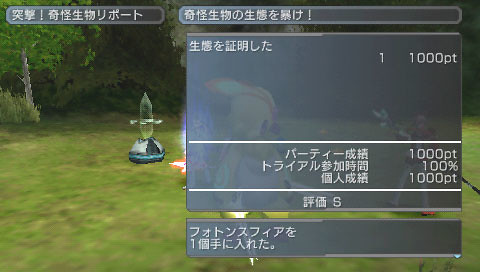The image appears to be a screenshot from an unidentified video game, set against a backdrop featuring a green lawn and a few trees. Dominating the right side of the image is a prominent black box displaying "1,000 points", with additional text stating "1,000 points 100% 1,000 points" beneath it. The text is written in either Chinese or Japanese, though its exact meaning is unclear. In the upper left corner, there is a smaller black box containing white Asian characters. The overall color palette consists predominately of muted gray and white tones, with occasional green hues in the background. Some characters are partially obscured by the interface elements, hinting at active gameplay.